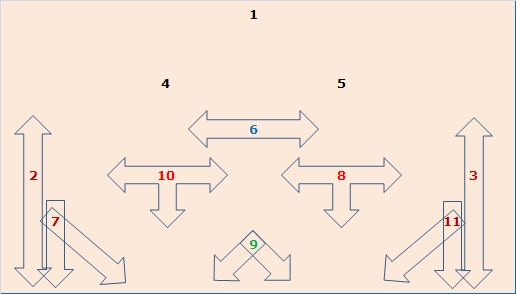The image showcases a vibrant and intricate geometric landscape with a predominantly pink and orange background. Dominating the scene are numerous thick arrow outlines oriented in various directions—vertically, horizontally, and diagonally. Each of these arrows either features double-ended points or single-ended tips, containing a distinct number, all rendered in different colors such as blue, red, and green.

At the very top of the image, a triangle composed of three numbers—`1` at the pinnacle, `4` in the bottom-left corner, and `5` in the bottom-right corner—sets the stage for the symmetrical design below. Flanking the extreme left and right sides are vertical, double-ended arrows, marked with the numbers `2` and `3` respectively.

Embedded within this symmetrical framework, a variety of other arrows are strategically placed, enhancing the complexity of the design. To the left of each of the vertically aligned double-ended arrows are single-ended arrows pointing downward. Diagonally aligned arrows emanate from these downward-pointing arrows, converging towards the center of the composition.

In the central region, horizontally oriented, double-ended arrows dominate the space. Some of these central arrows even feature additional arrows branching downward from their midpoints. Just above this central section sits another horizontal, double-ended arrow, prominently displaying the number `6`.

At the very bottom of the image, two interconnected diagonal arrows point in opposite directions, adding an additional layer of intricacy to the overall symmetrical pattern.

The exact meaning or intent behind the image remains unclear, but the meticulous arrangement of colorful numbers and directional arrows creates a visually compelling and harmoniously structured tableau.